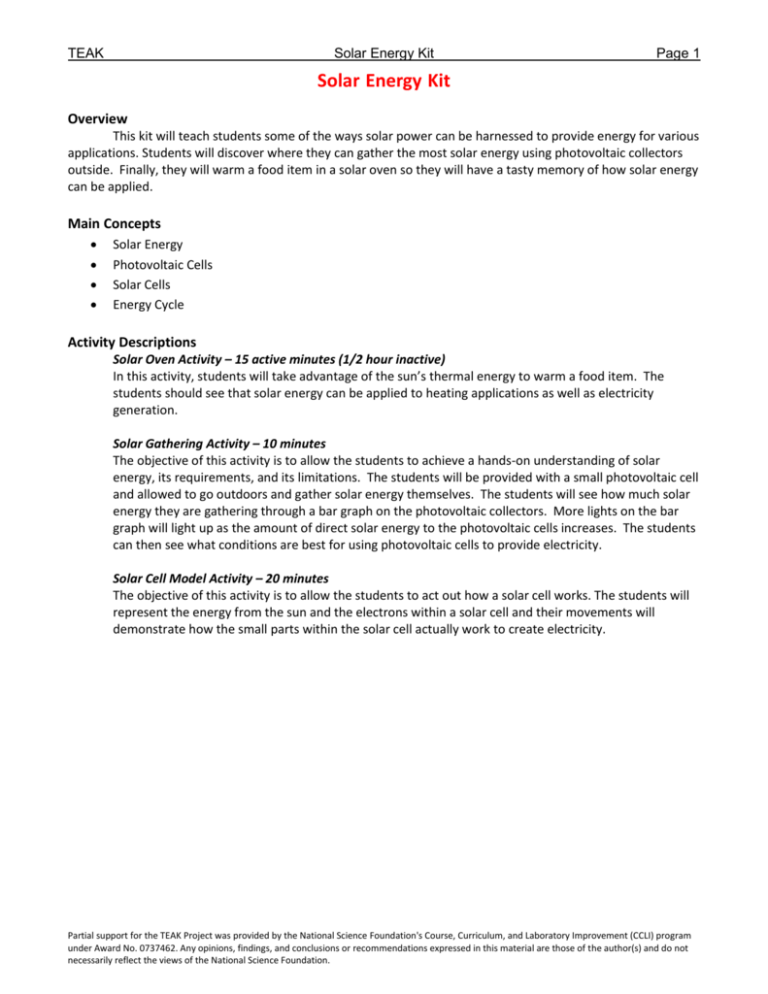The image features an educational document labeled "Solar Energy Kit." At the top middle, "Solar Energy Kit" is prominently displayed, with "Page 1" marked in the top right corner and the word "Teak" in the top left. Beneath these headings runs a black horizontal line across the width of the image. 

Just below this line, the title "Solar Energy Kit" appears again, but this time bolder and in red text. Directly below this, on the left side, the word "Overview" is highlighted in bold black text. The overview reads: "This kit will teach students some of the ways solar power can be harnessed to provide energy for various applications. Students will discover where they can gather the most solar energy using photovoltaic collectors outside. Finally, they will warm a food item in the solar oven so they will have a tasty memory of how solar energy can be applied."

Further down on the left, the section "Main Concepts" is clearly marked, listing four key points: 1) Solar Energy, 2) Photovoltaic Cells, 3) Solar Cells, and 4) Energy Cycle. 

Directly beneath this section, "Activity Descriptions" is labeled, followed by three specific activities outlined for students: 1) Solar Oven Activity, 2) Solar Gathering Activity, and 3) Solar Cell Model Activity.